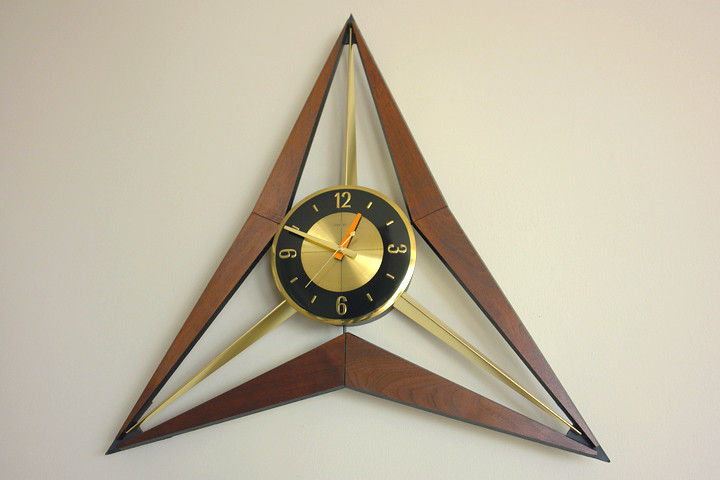This photograph features a striking mid-century vintage wall clock, evocative of the 1950s or 1960s era. The clock boasts a unique starburst design, reminiscent of the Star Trek insignia. Its distinctive frame takes the form of a somewhat warped triangle, with brass rods extending from each angle, reinforcing its star-like appearance. This brass coloring, with a yellowish tint, is prominent throughout the clock’s exterior.

The outer frame of the clock combines wood and steel, with a wooden outline that seamlessly integrates into metal panelling, exuding an elegant, brassy gold finish. At the center of the frame lies the circular clock face, which is primarily black with golden and orange details. The clock features only four numerals—12, 3, 6, and 9—while the remaining hours are marked by minimalist notches.

The hands of the clock are brass, with the hour hand in vibrant orange and the minute and second hands in gold. The non-digital, mechanically-operated clock currently displays the time at approximately 12:49. The white wall backdrop accentuates the clock’s vintage charm and intricate construction.